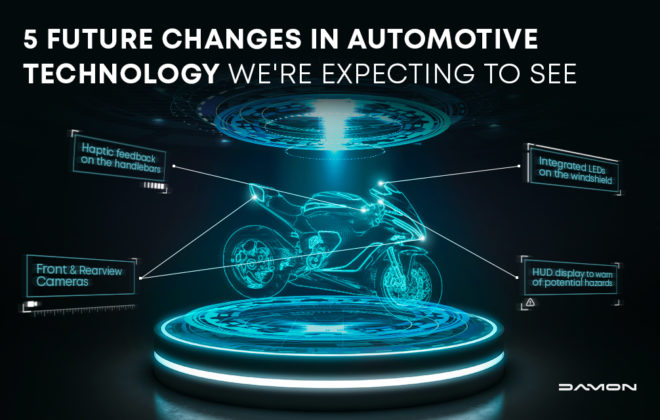In the center of this black poster, which spans roughly 1.5 times wider than it is tall, there is a striking, computer-generated visual display. The top of the poster features the white text, "Five Future Changes in Automotive Technology We're Expecting to See." Below this text, a cylindrical platform emits various hues of white and teal light, creating a futuristic, digital ambiance. Hovering above the platform is a translucent, teal-hued hologram depicting a motorcycle. Positioned around the motorcycle are several white lines connecting to turquoise boxes, each highlighting key innovative features. These include integrated LEDs on the windshield, front and rear-view cameras, haptic feedback on the handlebars, and a HUD display. The bottom right corner of the poster features the company name, "D-A-M-O-N." The entire scene is set against a stark black background, emphasizing the illuminated elements and giving the overall composition a dynamic, cutting-edge appearance.